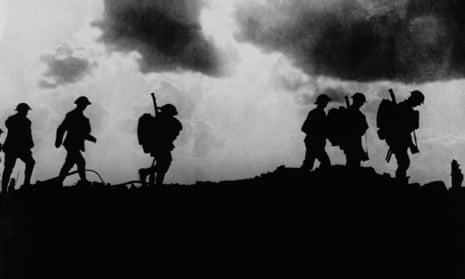This is a small, stark black and white rectangular photograph likely from World War I, depicting six soldiers in silhouette marching from left to right across a jagged, black hill that sits just below the midpoint of the image. The soldiers are arranged with three on the left half, spaced further apart from each other, and three on the right half, positioned closer together. Notably, three of the soldiers are carrying large backpacks. They are all wearing doughboy helmets, characteristic of World War I. Behind the soldiers, the sky is bright and cloudy, filled with smoke that darkens towards the top right corner, giving the scene a dramatic, almost apocalyptic atmosphere. The horizon line created by the hill rises slightly towards the right before dipping again at the right edge, and the ground beneath the soldiers is completely black, devoid of any detail, enhancing the stark contrast of the image.